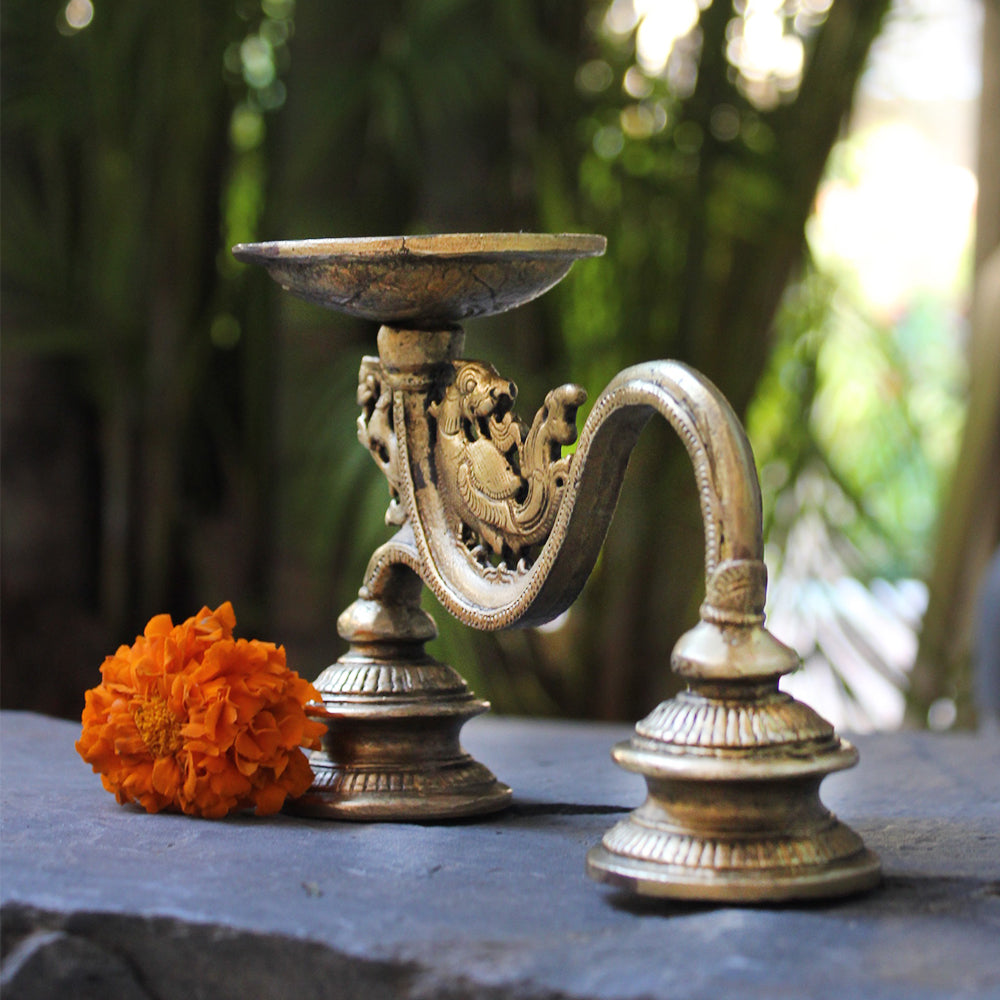This is a detailed color photograph showcasing an intricate, brass candle holder with an ornate design. The candle holder, which appears to have a dragon motif and sloping, rope-like imagery, features two curved legs standing on a dark stone bench or table. At the top, a gold-colored saucer, potentially to hold a candle and capture melted wax, is intricately etched and slightly cracked, supported by two antique brass knobs at the base. Next to the candle holder is a striking orange pom-pom-like flower, without leaves, adding a vibrant contrast. The background of the image is out of focus, revealing a lush green landscape with light filtering through, possibly indicating a forest or dense foliage, with sunlight casting shadows from the left. The entire composition emphasizes the ornate brass fixture and the bright flower against the serene, blurred greenery.